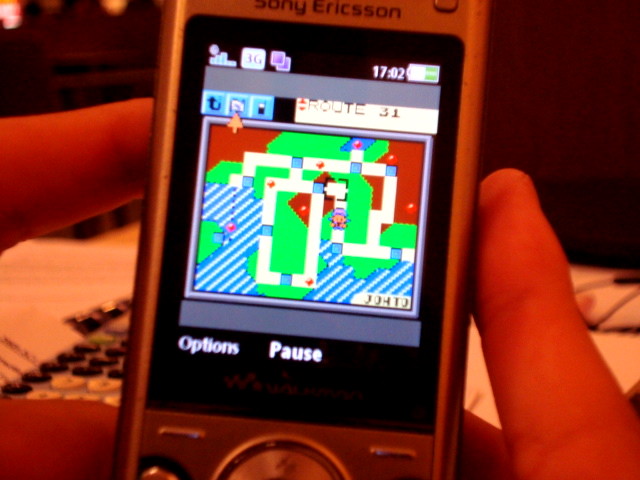In this detailed photograph, we see a classic Sony Ericsson cell phone, reminiscent of the early 2000s. The phone's screen prominently displays an engaging game of Pokémon, featuring charming 90s-style pixel art. Central to the screen, there is a map labeled "ROUTE 31," showcasing a character walking along a path. The map is detailed with water bodies, grassy areas, and multiple pathways available for exploration. The interface includes various game controls such as options and pause buttons, along with small icons that enhance the gaming experience.

Positioned at the top of the phone's screen is a status bar indicating the phone's battery level and other functional icons. The user's fingers, appearing light-skinned, firmly grasp the device, with three fingers visible in the shot. In the background, there's a blurred room setting with a discernible dark wall and a hint of the user’s clothing, which is a light blue outfit. The softness of the out-of-focus background accentuates the nostalgic focus on the vintage phone and classic game.